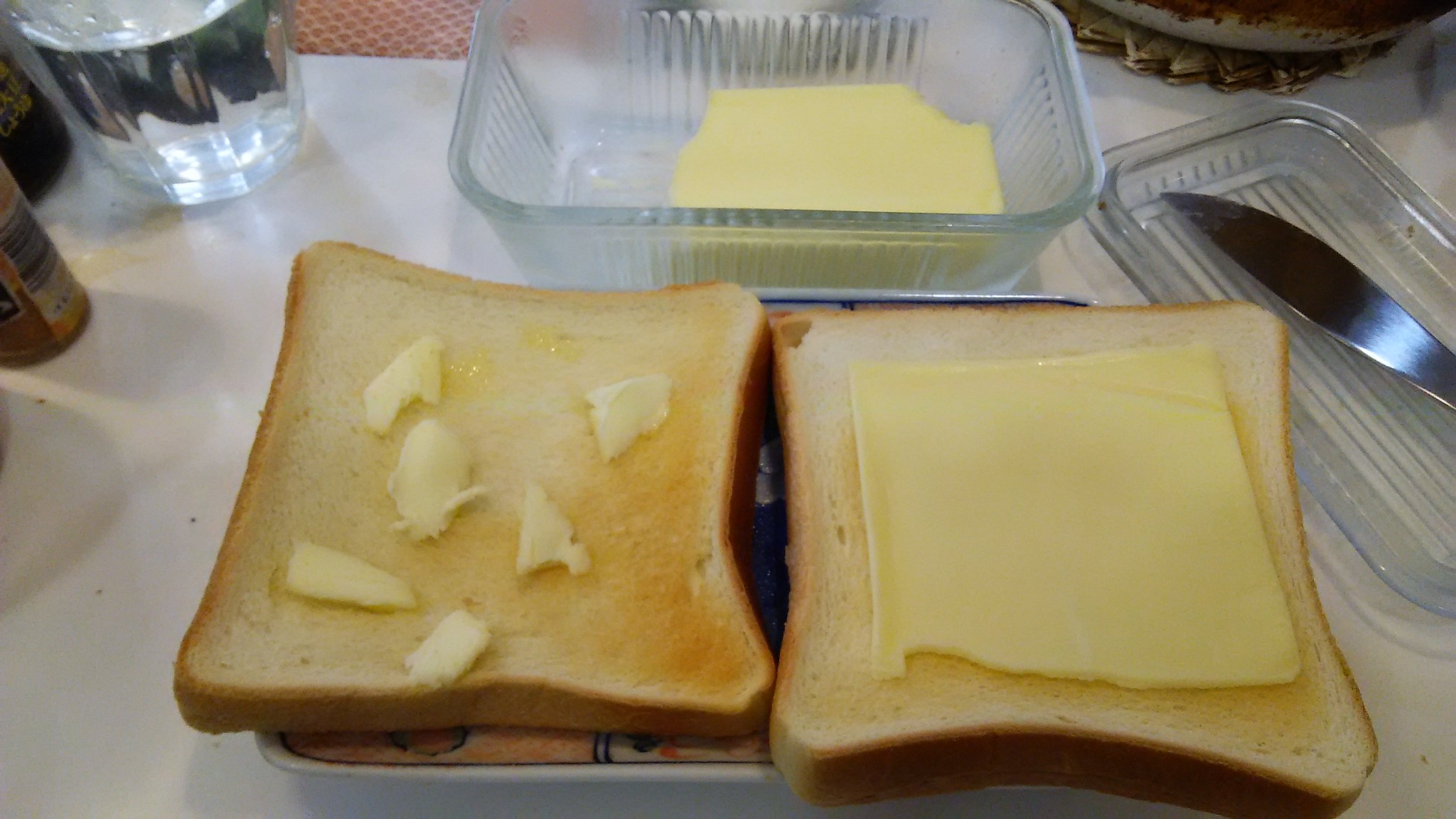In this close-up photograph, two pieces of toasted white bread sit on a vibrant plate with yellow and orange tones, partially obscured by the bread. The left slice features six irregularly shaped pats of butter, beginning to melt into the toast's surface. Meanwhile, the right slice is topped with a thin, torn slice of white American processed cheese. In the background, a clear glass butter dish containing a partially used stick of butter stands out, with its lid placed to the right bearing a table knife. A clear glass of water and a small bottle are visible in the upper left corner. The setting is a white table, possibly covered by a flawlessly taut tablecloth, adding to the image's overall crispness.